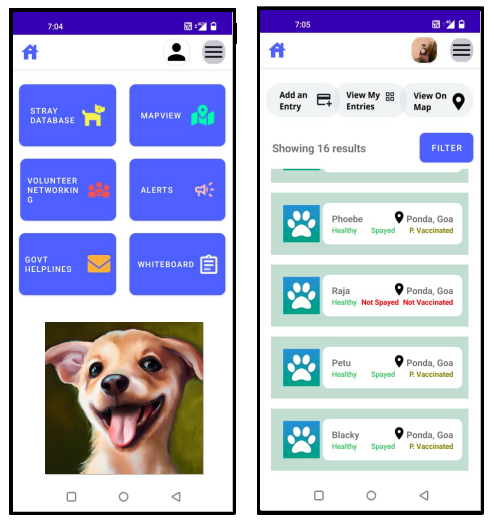Here's a cleaned-up and detailed caption for the image:

---

The screenshot displays a webpage with a clean and organized design. At the top of the page, there is a royal blue banner featuring three icons: a home, a person, and three horizontal lines. Below this banner, the main content area is set against a white background and contains six blue boxes arranged in two rows.

Each box has a title in white text accompanied by an icon:
1. "Stray Database" with a dog icon.
2. "Map View" with a map icon.
3. "Volunteer Networking" with red icons of people.
4. "Alerts" with a pink megaphone icon.
5. "Government Helpline" with a yellow envelope icon.
6. "Whiteboard" with a clipboard icon.

Below these boxes, there is an image of a dog with its mouth open, rendered to look like a painted but computer-generated picture. Further down, there are interactive elements: a circle, a square, and an arrow, which allow users to choose different options. When clicked, these options open up different pages where users can view rescue pups available for adoption, add new entries, view their own entries, or check the location of entries on a map.